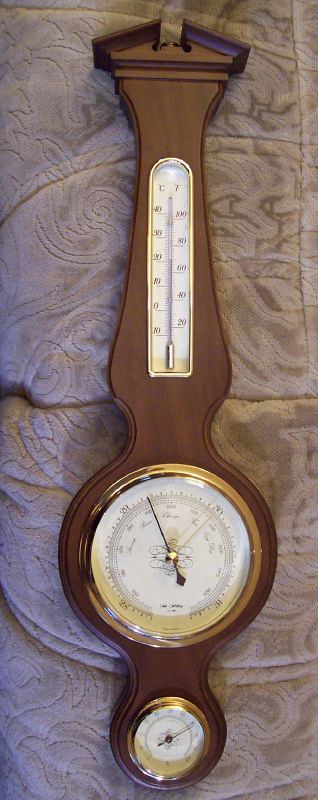A beautifully intricate, colonial-style clock is displayed prominently in this image. The clock features three distinct sections: a clock face, a thermometer, and possibly a calendar. Crafted with exquisite attention to detail, the clock boasts intricately carved wooden elements with chamfered edges and a sophisticated brass frame encircling each of the clock's components. The clock and its accessories are resting on a textured surface that appears to be either a couch or a blanket, characterized by an embroidered, fuzzy gray fabric. Natural light from a nearby window illuminates the scene, adding a balanced warmth to the overall composition without overpowering the intricate details of the clock.